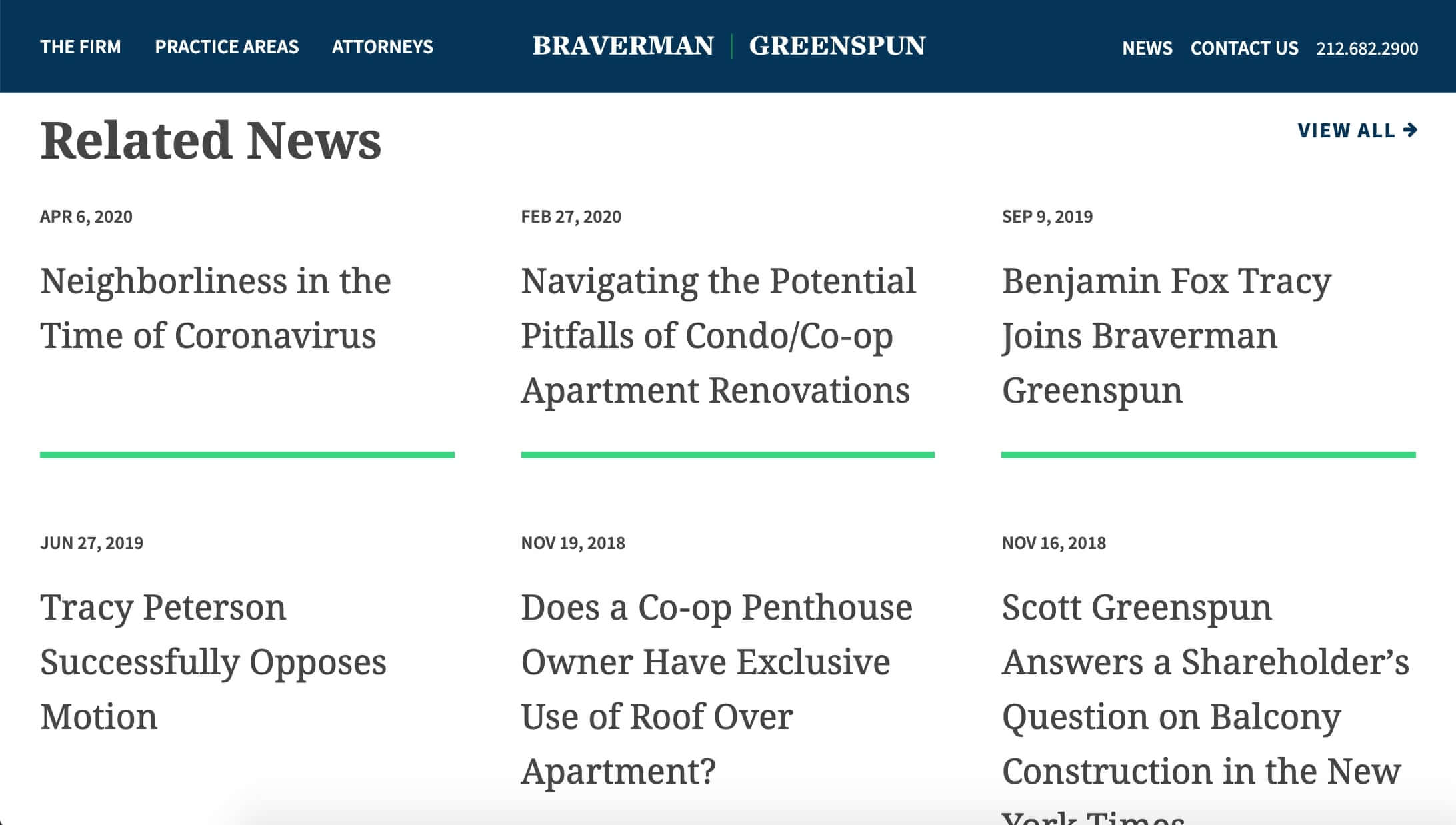This appears to be a screenshot of a webpage for the law firm Braveman-Greenspun. At the top of the page, there is a blue navigation bar with white text that reads "The Firm," "Practice Areas," and "Attorneys" from left to right. In the center of the bar is the firm's name, "Braveman-Greenspun," and to the right, there are links for "News," "Contact Us," and a phone number, 212.682.2900, all in white text.

Beneath the navigation bar is a large white section titled "Related News" in prominent black text. To the far right of this title, there is a "View All" option in blue text accompanied by a right-pointing arrow. This section contains six news articles arranged in two rows and three columns. Each article has a date at the top, followed by the title:

- **Top Left:** "April 6, 2002 - Neighborless in the Time of Coronavirus"
- **Top Center:** "February 27, 2022 - Navigating the Political Pitfalls of Condo Co-op Apartment Renovations"
- **Top Right:** "September 6, 2019 - Benjamin Fox Tracy Joins Braveman-Greenspun"

- **Bottom Left:** "June 27, 2009 - Tracy Pearson Successfully Opens Motion"
- **Bottom Center:** "November 19, 2018 - Does a Co-op Penthouse Owner Have Exclusive Use of Roof of Their Apartment?"
- **Bottom Right:** "November 16, 2018 - Scott Pearson Answers a Shareholder's Question on Balcony Construction in The New York Times"